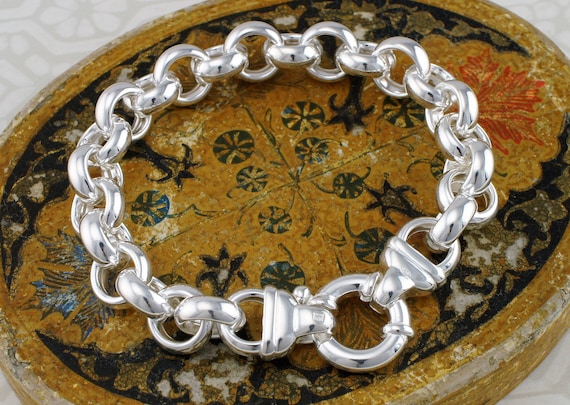The image prominently features a highly polished, glistening silver chain bracelet with interlocking links and a clasp. This central silver chain is placed atop a worn, oval-shaped, possibly antique storage box, which is golden-rod or tannish in color. The box bears intricate floral and leaf designs in blue, gold, and black, with a notable red leaf detail at the top. The vibrant bracelet starkly contrasts with the box’s aged appearance. The entire setup rests on a surface with a marble-like flower design in gray, indicating it might be a counter or table, adding to the composition's depth. The background is a light color with faint designs, situating the scene in what appears to be an indoor environment.